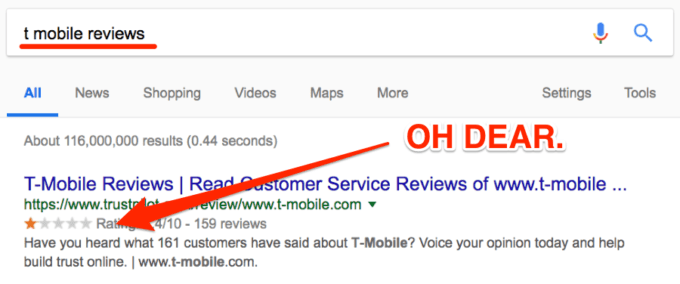The screen capture showcases a Google search results page for "T-Mobile reviews." At the top, the white search box prominently displays "T-Mobile reviews" in black font, accompanied by a distinctive red line below. Inside the search box, recognizable icons such as a blue, red, and gold microphone and a blue magnifying glass are visible. Just beneath the search box, a menu bar appears, featuring categories like "All" (highlighted in blue), "News," "Shopping," "Videos," "Maps," "More," "Settings," and "Tools," all in gray.

Further down, the search results section begins, displaying the number of results and the duration of the search. Notably, there is bold red text that reads "OH DEAR." A prominent red arrow points to a rating featuring one gold star, indicating customer dissatisfaction with T-Mobile on Trustpilot. The search result for T-Mobile reviews is highlighted in blue and reads, "T-Mobile reviews read customer service reviews www.t-mobile." Adjacent to this, there's a green Trustpilot badge, reinforcing the connection. The red arrow further draws attention to the dismal one-star rating based on 159 reviews. Additionally, a call to action below asks, "Have you heard what 161 customers have said about T-Mobile? Voice your opinion today and help build trust online www.t-mobile.com."